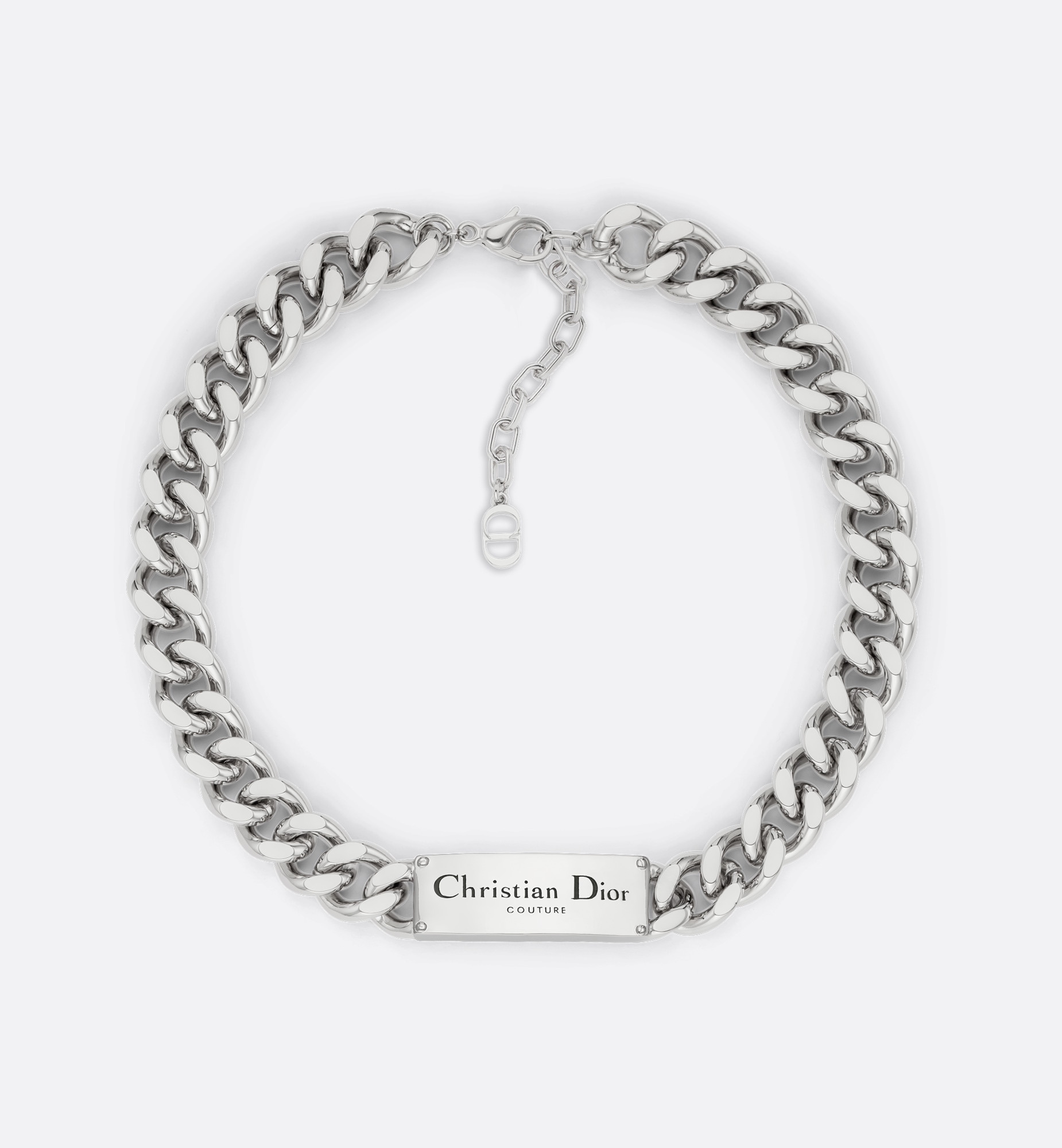This is an image of a silver metallic choker necklace, prominently featuring a Christian Dior Couture brand plate at the center front. The picture, likely intended for a product listing, is expertly lit and focused, suggesting it was taken in a light box against a pure white background. The necklace showcases a design of large interlocked links, which somewhat resemble a herringbone pattern, lending it an intricate and elegant appearance. The clasp features a small tail chain that dangles, adding a delicate touch and making it easy to identify the back of the necklace. This detailed and stylish piece is clearly intended for women's fashion.